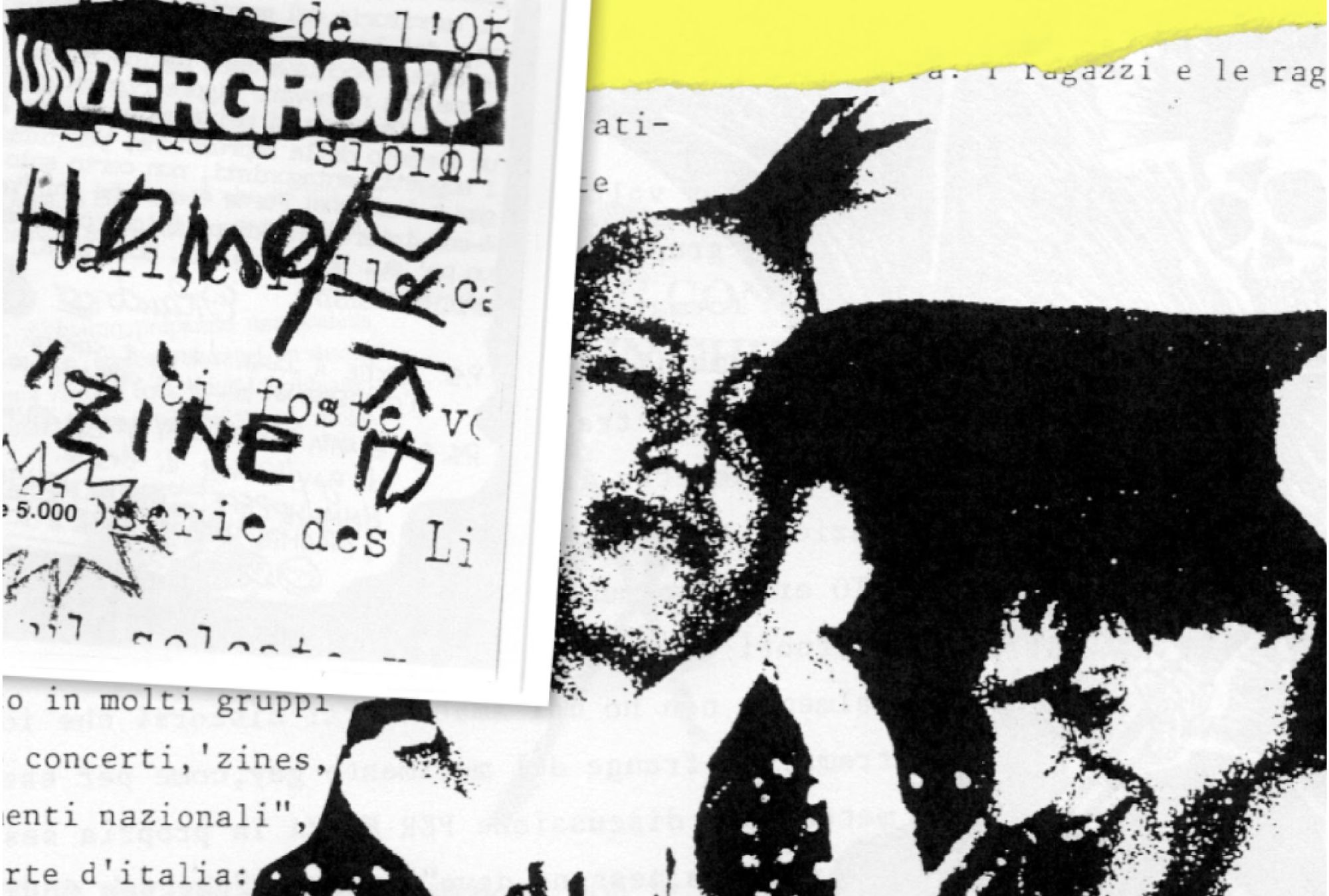The image is a detailed, black-and-white collage featuring a variety of overlaid documents and photographs, dominated by a central theme of underground home and culture. At the top of the image, there's a noticeable section of yellow that extends from the middle to the right, covering some of the text and paper underneath. The predominant element in the image is a black-and-white photograph that showcases two men: the one in the center with a tall mohawk hairstyle has a neutral expression, while the man to his right, wearing a large cap, is smiling. The photograph is somewhat blurry and has a pointillist quality. To the left of this main photo is a significant amount of foreign text, possibly Italian, which includes the word "underground" prominently written in black at the top left. The various documents and pieces of paper appear torn and layered, with partial texts visible throughout, adding to the collage's fragmented and dynamic appearance.